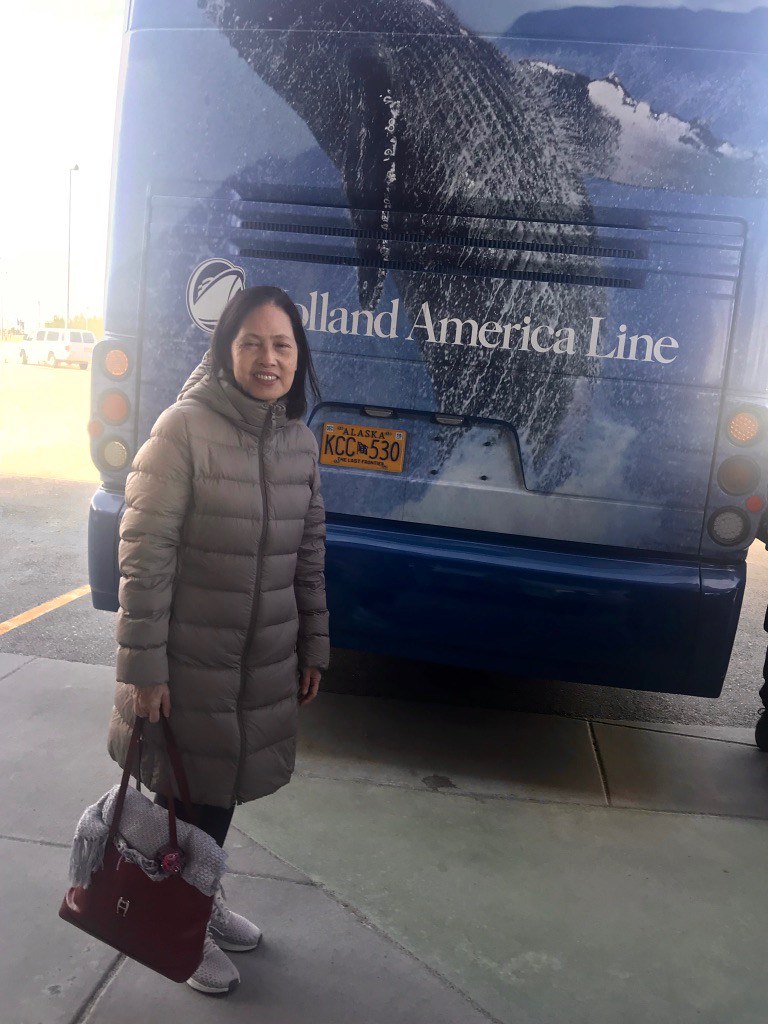In this image, an older Asian woman with shoulder-length black hair smiles warmly at the camera while standing in front of a large, blue Holland America Line tour bus. She is dressed for cold weather in a long, gray puffy jacket, black pants, and white sneakers. Her attire reflects a practical yet cozy style, akin to what one might expect from someone accustomed to colder climates, such as Canada. In her hand, she carries a dark red leather tote bag with a gray scarf neatly rolled between its handles. Behind her, the bus's rear is adorned with a vivid mural of a whale breaching the water, adding a dynamic and lively backdrop to the scene. The bus sports a yellow Alaska license plate with the numbers KCC 530, grounding the image in a specific locale. In the distant background, a parking lot with a van and a light post can be seen, completing the scene.